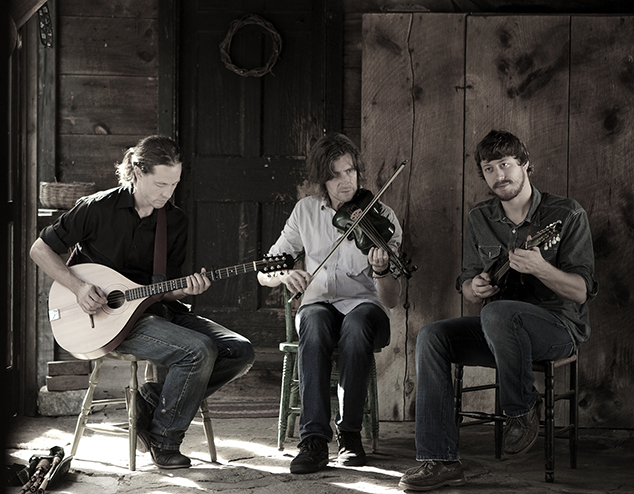In this evocative black-and-white photo, three male musicians, appearing to be in their late twenties, are seated on wooden chairs on a rustic porch, which could either be inside or outside an old wooden cabin with weathered, plank walls. The musician on the left, with his hair pulled back in a ponytail, appears to be playing a lute or possibly a mandolin. The central figure, with long flowing hair, is engaged in playing a violin. Meanwhile, the musician on the right, distinguished by his beard and mustache, is strumming what looks like a mandolin or a ukulele. A dry twig wreath adorns the large wooden door behind them, adding to the western, rustic ambiance. Sunbeams penetrate from the left side, casting illuminated patterns on the porch boards. All three wear jeans and casual dress shirts, absorbed in their performance, capturing a serene moment of artistic camaraderie.